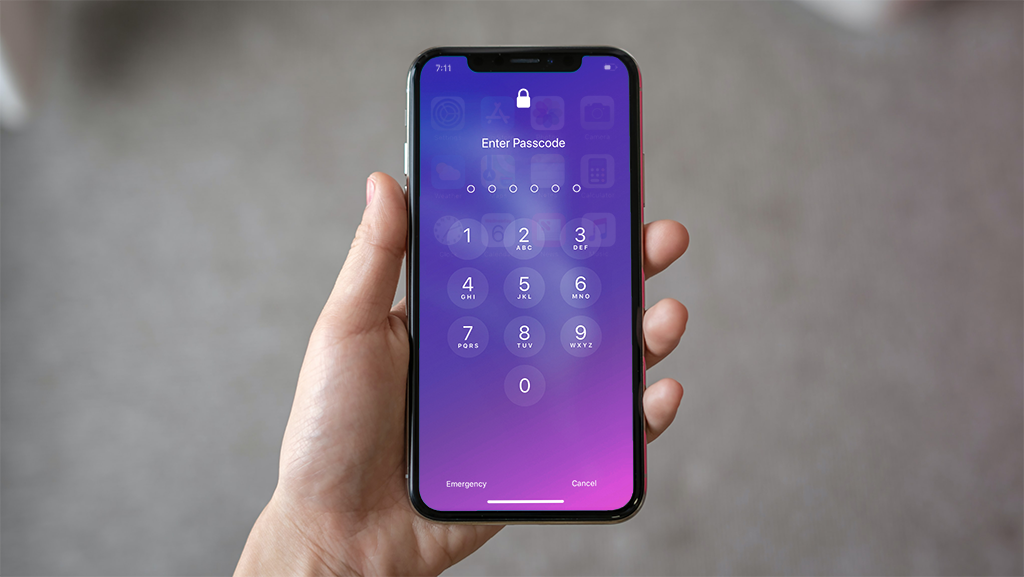The image showcases a detailed close-up of a hand holding a black iPhone, distinguishable as a newer model without a home button. The iPhone's screen displays the lock screen with a prompt to enter a six-digit passcode, accompanied by a lock symbol above the text "Enter Passcode." The numeric keypad from 0 to 9 is clearly visible below, along with options for emergency call and cancel. The time displayed on the phone is 7:11. The blurred gray background contrasts with the focus on the hand and device, while the phone's wallpaper features an ombre gradient transitioning from purple to pink. The hand, without any nail polish, shows the side of the thumb, the bottom of the palm, and three fingertips peeking from the right side of the phone. The home screen visible behind the keypad indicates only the default apps are installed, reflecting a typical uncustomized setup.